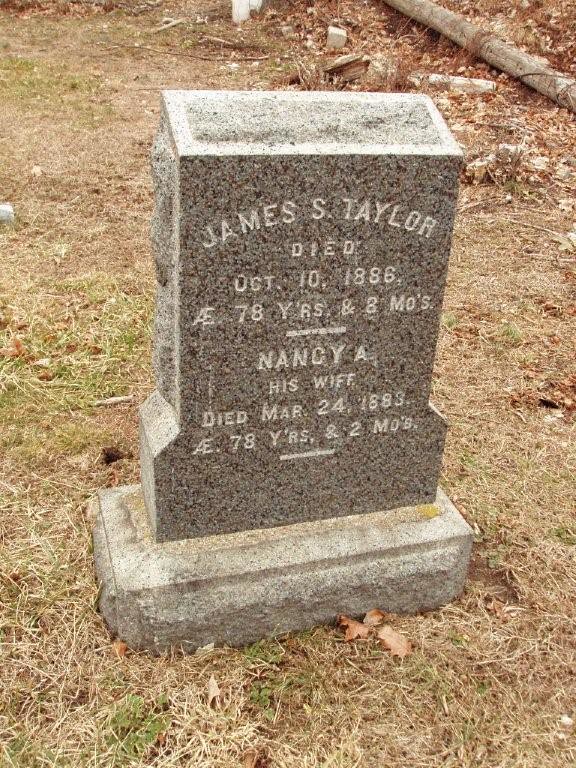The image depicts a tall, granite gray tombstone set in an outdoor area that appears to be a cemetery in the fall. The ground is covered mostly with dead grass, interspersed with a few patches of green. The tombstone is situated on a rectangular concrete base, surrounded by dead leaves and debris. In the upper portion of the image, there's a fallen tree branch adding to the scene of decay. The tombstone is the central focus, with its light gray surface etched in white letters, reading: "James S. Taylor, died October 10, 1886, aged 78 years and 8 months." Below, in a similar inscription, it commemorates "Nancy A., his wife, died March 24, 1883, aged 78 years and 2 months." The tombstone is solitary, with no other headstones visible in the frame.